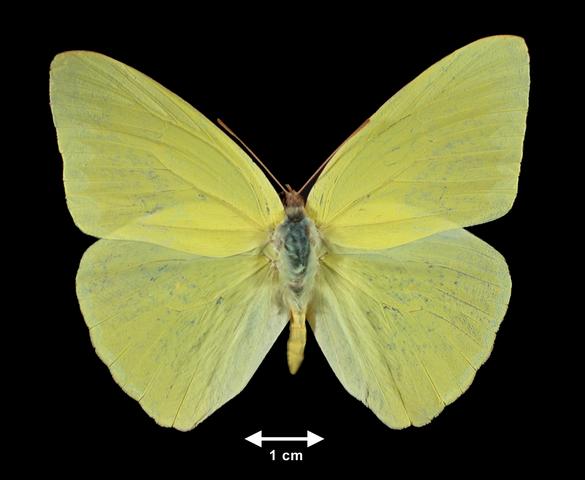This image features a yellow moth prominently displayed against a stark black background, allowing for intricate details to be clearly visible. The moth's four wings—two at the top and two at the bottom—are fully extended, showcasing the delicate veins and lines that run through them. In the center, the moth's body is visible, appearing fuzzy and predominantly gray with a mix of beige and yellow hues. The moth's antennae, which are brown and slightly curved, extend from the top of its head. A measurement indicator with arrows pointing left and right denotes a scale of 1 centimeter, providing a reference for the moth's size. The tail end of the moth tapers off into a slightly skinnier, less fuzzy section compared to the central area.